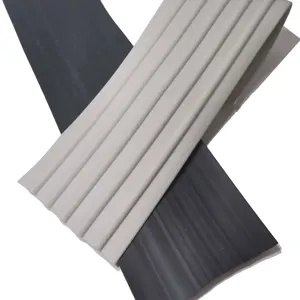The image depicts a detailed illustration of two rectangular pieces, each with distinctive textural and color characteristics. The bottom piece is a black rectangle with subtle vertical white streaks that create a shaded effect primarily towards the lower left corner. These streaks are less pronounced compared to those on the top piece. The top rectangle, lying diagonally from the upper right to the lower left, is gray with prominent vertical stripes. These stripes, darker than the gray background, give the piece a ribbed or pleated appearance, suggesting that they would be tactile if touched. Together, the black rectangle serves as a backdrop, with its muted streaks providing a contrasting foundation to the more textured and visually striking gray rectangle above it.